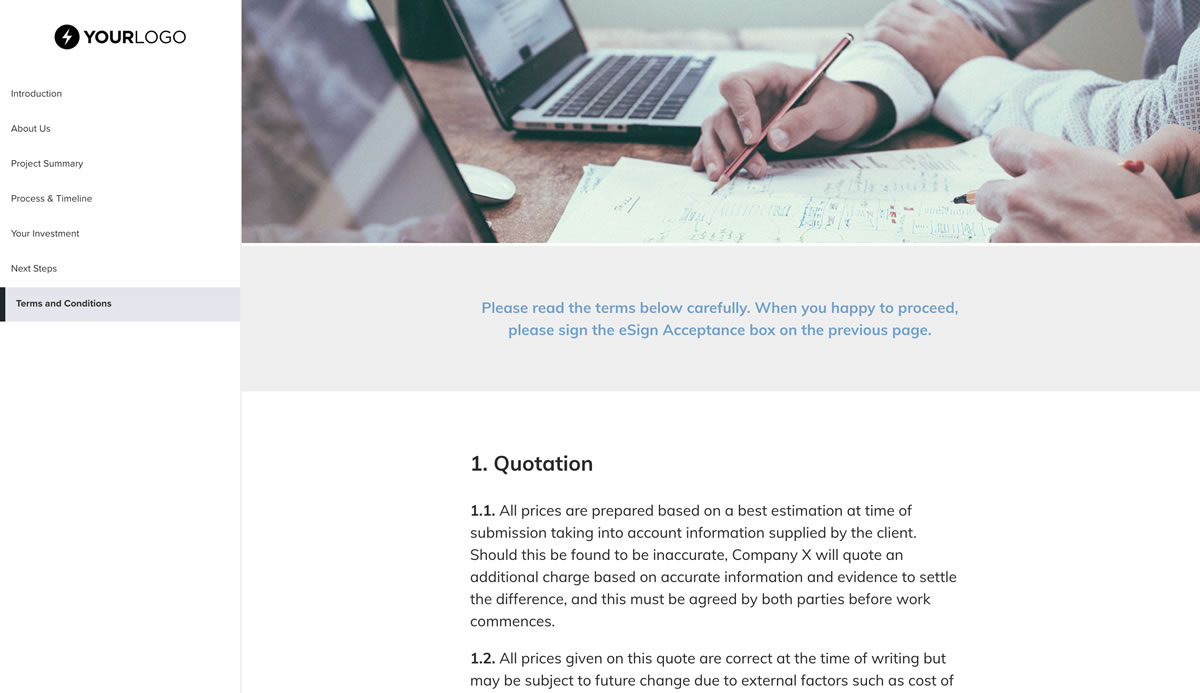The webpage is a professional design platform dedicated to logo creation, prominently branded with an eye-catching logo located in the upper left corner—a bold black circle featuring a white lightning bolt. The heading 'Your Logo' is presented with 'Your' in bold black lettering and 'Logo' in standard black script.

On the left-hand side of the screen, a navigation menu provides essential links: 'Introduction,' 'About Us,' 'Project Summary,' 'Process and Timeline,' 'Your Investment,' 'Next Steps,' and the currently selected 'Terms and Conditions.'

At the top of the page, a visually engaging image displays two laptops and four hands collaboratively working on mathematical documents. Below this image, a highlighted light gray section with code-blue text commands reader attention: "Please read the terms below carefully. When you're happy to proceed, please sign the e-sign acceptance box on the previous page."

The terms and conditions are meticulously detailed in a user-friendly format, featuring bold numbered headings for clear reference. It starts with:

1. "All prices are prepared based on estimates at time of submission, taking into account information supplied by the client. Should inaccuracies be found, Company X will quote an additional charge based on accurate information and evidence to settle the difference. This must be agreed upon by both parties before work commences."
2. "All prices given in this quote are correct at the time of writing, but may be subject to future change due to external factors such as cost of..." (The sentence cuts off here).

The entire terms and conditions section is laid out in black text against a stark white background, ensuring readability and seriousness. The rest of the page mirrors the brand’s ethos—minimalistic yet professional, leveraging primarily white and light gray backgrounds complemented by black and grayscale typography. The aesthetic and functional choices indicate a focus on clarity and ease of navigation, enhanced by the striking logo that symbolizes creativity and precision in logo design services.